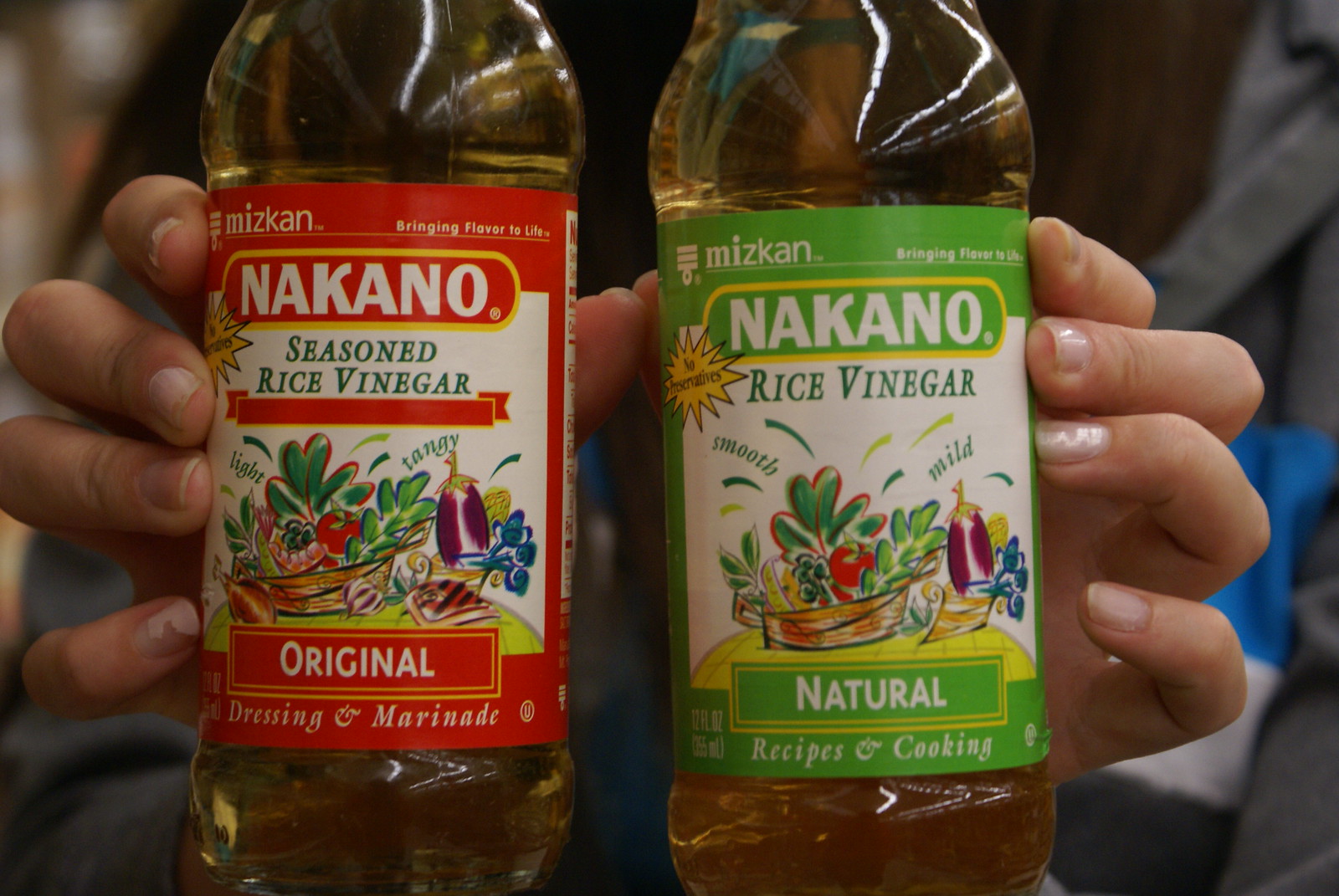In the photograph, a person is holding up two glass bottles, each prominently labeled. The bottle in their right hand, positioned on the left side of the image, features a red and white label that reads "Nakano Seasoned Rice Vinegar." At the bottom of this label, it is marked with "Original Formula," and beneath that, the words "Dressing and Marinade" are clearly visible. The bottle in their left hand, seen on the right side of the image, has a green and white label. This label is largely identical to the first, except it reads "Rice Vinegar" instead of "Seasoned Rice Vinegar." Additionally, where the first bottle mentions "Original," this one states "Natural." Finally, the text at the bottom of this label reads "Recipes and Cooking" rather than "Dressing and Marinade."